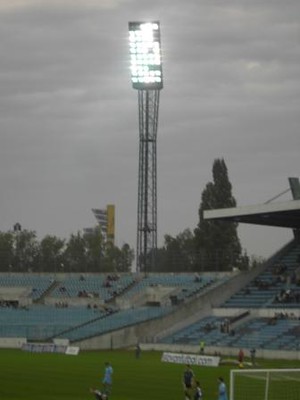The image depicts a soccer stadium late in the day, enveloped in a sad, gray, and very cloudy sky. Dominating the scene is a towering wireframe light tower, intricately designed with what seems to be at least 50 smaller floodlights, some of which are lit, forming a pattern that bears a slight resemblance to a Pac-Man face. The light tower starts from behind the stadium and stretches up to the top of the image, casting a bright illumination on the field below.

The stadium’s stands, though washed-out and somewhat dirty, feature light blue seats with a smattering of spectators. The structure itself appears to be made of a blue and beige-white stone material. The lush, lime-green grass on the field contrasts with the otherwise dreary atmosphere. A soccer goal is visible at the bottom right corner of the image, alongside a net strung between poles.

In the foreground, a few people can be seen milling about on the field, while tall trees rise behind the stadium, framing the scene. The presence of these scattered individuals and the lightly populated stands add a sense of tranquility to the image as night approaches and the artificial lights prepare to take over the diminishing natural light.